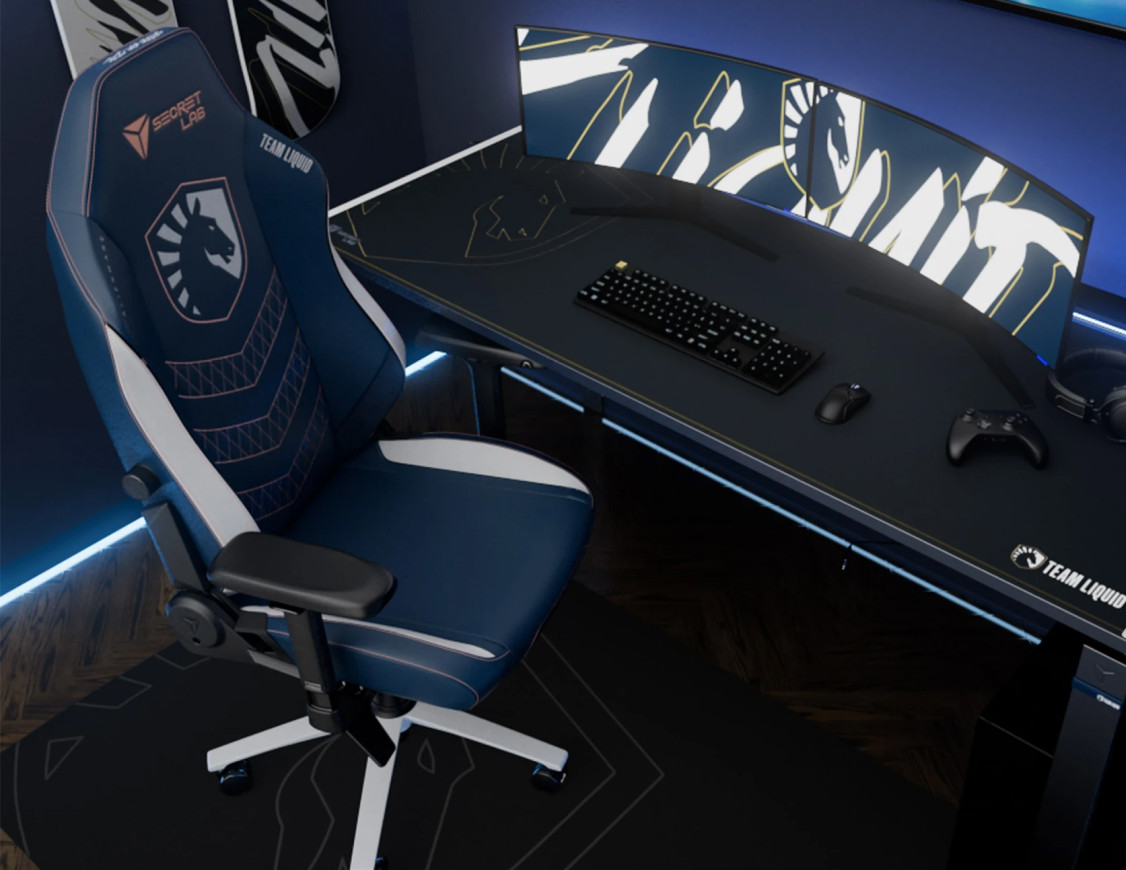The image features an organized and immersive PC gaming setup. At its center is a sleek, dark blue gaming desk, emblazoned with the Team Liquid logo - a horse within a shield - in the bottom right corner. This emblem is consistently repeated throughout the setup, appearing on the desktop screens, the ergonomic gaming chair with white and gray accents, and even on the floor mat beneath the chair. The chair, prominently branded by Secret Lab, offers substantial support with armrests and enhances the gaming experience. The desk is equipped with essential peripherals, including a keyboard, mouse, game controller, and headphones. The dual monitor setup, featuring two wide, flat screens, also displays the distinctive Team Liquid logo. Completing the room's cohesive and modern aesthetic, neon lighting along the floor adds a vibrant, immersive ambiance, perfect for dedicated gaming.